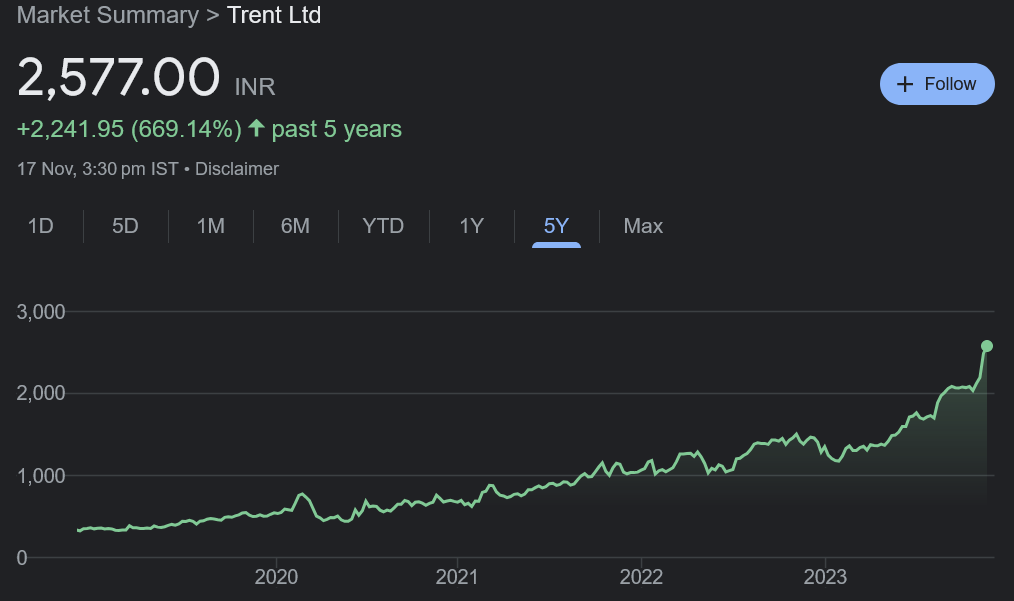**Detailed Caption for the Stock Market Chart of Trent Limited:**

The image showcases a detailed stock market chart for Trent Limited. In the top left corner, "Market Summary" is prominently displayed, accompanied by an arrow pointing to the company's name, Trent LTD. The current stock price is clearly indicated in large numerals as 2577 INR. Directly beneath this, the chart highlights an impressive 5-year performance, showing a substantial increase of 2,241.95 INR, which equates to an exceptional 669.14% rise over the period.

The data was last retrieved on the 17th of November at 3:30 p.m. IST, ensuring the figures are up-to-date. Below the performance metrics, there are multiple options to view the stock's historical data over various time horizons, ranging from one day to the maximum available timeframe. 

The main stock chart provides a visual representation from 2019 up to the present, November 2023. The trend line reveals significant upward movement with intermittent periods of volatility, suggesting an overall positive growth trajectory for Trent Limited's stock.